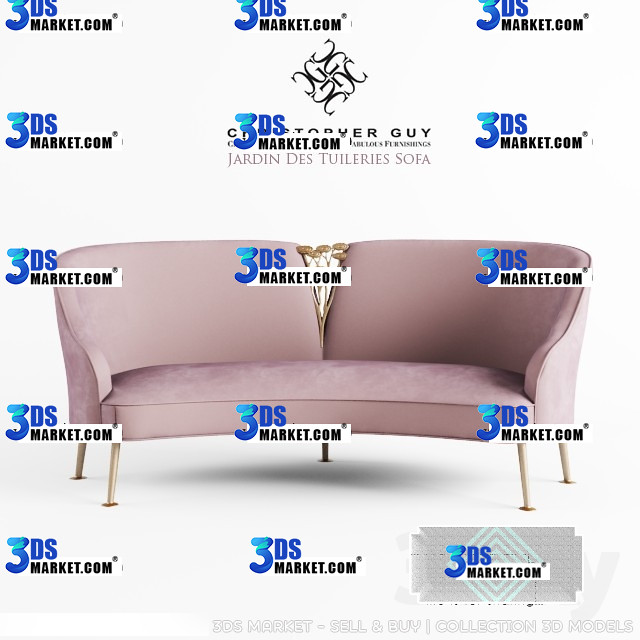The image features a detailed advertisement for 3dsmarket.com, showcasing a mid-century modern loveseat known as the Jardin des Tuileries Sofa. This elegant piece, with its curved armrests and back, is displayed prominently against a pristine white background, accentuated by a slight shadow beneath. The sofa, which comes in a reddish-gray to light pink-purple hue, sits on five slender legs, adding to its sophisticated design. Across the entire image, there is a noticeable watermark of 3dsmarket.com, with "3ds" in blue and "market.com" in a smaller black font, repeated throughout. At the bottom, amidst multiple watermarks, there is text promoting 3dsmarket’s collection of buy-and-sell, 3D models. The sofa's name, Jardin des Tuileries, is elegantly displayed, indicating the exclusive design of this beautiful furnishing.